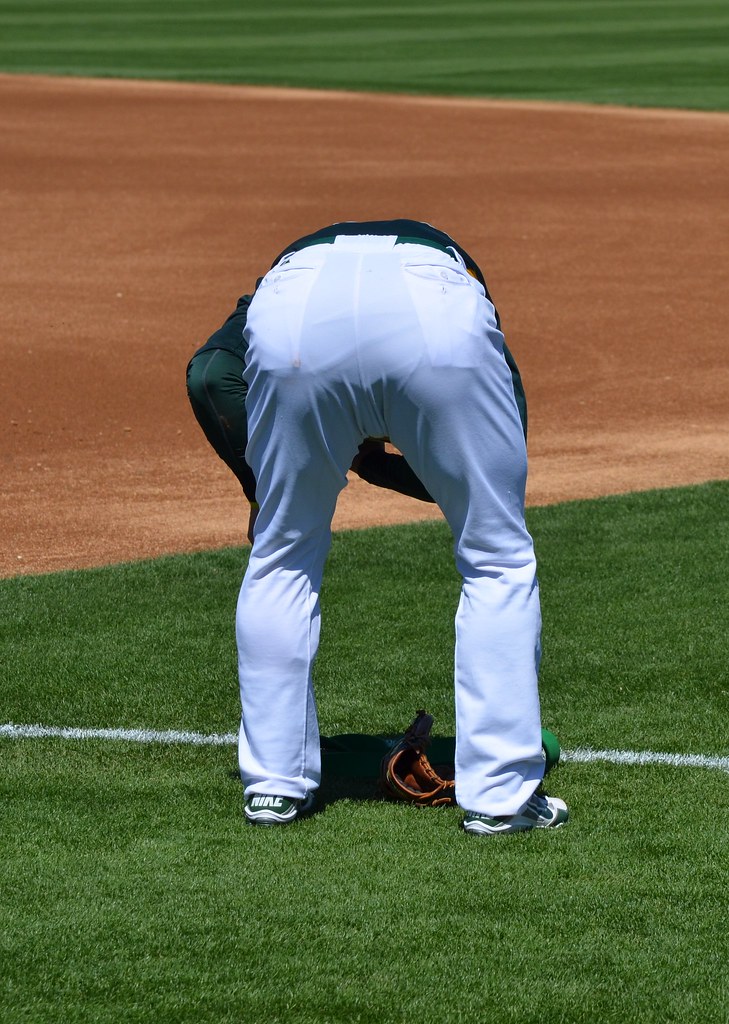In this rare daytime image taken on a well-manicured baseball field, a man is captured bent over with his back facing the camera. He is positioned on the green grass, near the first baseline, which features a clearly visible white line. The field exhibits a mixture of colors: green from the grass, white from the man's long pants, brown from the dirt infield, and orange and white from a helmet on the ground. He is wearing Nike sneakers, identifiable by the inscription on the back. His attire includes a green long-sleeve polo shirt. In front of him, positioned between his legs, is a brown baseball glove. To the right of the glove, another green item lies on the ground. The scene seems to capture a moment before the start of the game or after the field has been freshly maintained, as indicated by the pristine condition of the dirt infield and the groomed grass.